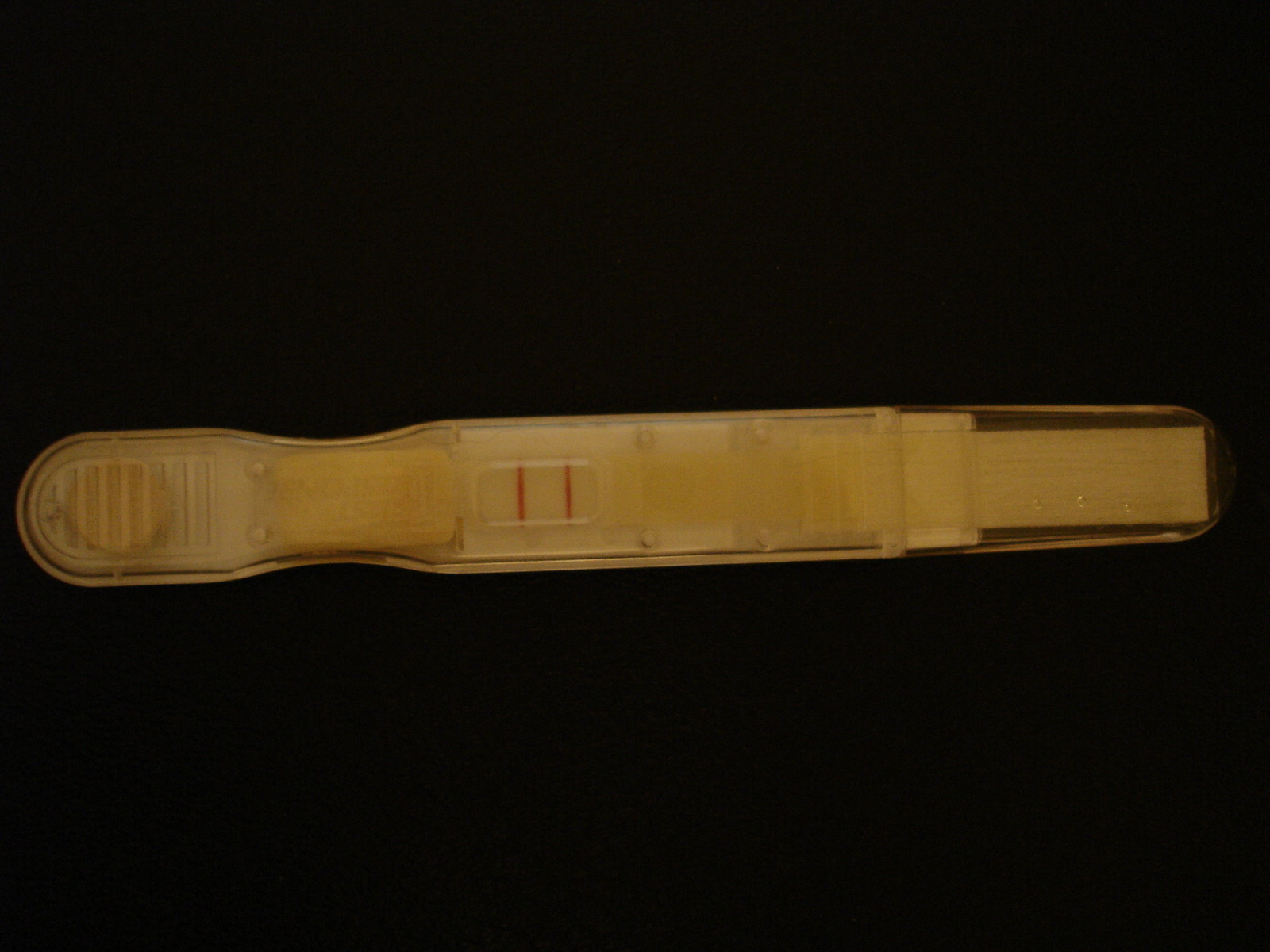The image displays a medical test stick set against a solid black background. The stick is primarily light brown in color and features a straight central section that tapers slightly to a rounded tip at one end and an indented area leading to a rounded end at the opposite side, resembling a small plastic cap. Along the light brown strip, there is a panel comprised of various components: a segment of brown plastic transitions into a section of white plastic, which houses a small display window with two red lines indicating the test results. Adjacent to the window is a yellowish pad designed for sample application. Further along the stick, there appears to be a button-like structure with textured lines, suggesting it could be pressed up or down, although it is all made of plastic and likely part of the device's design. The overall construction suggests ease of use, requiring just a small sample of blood, urine, or another bodily fluid to operate the test.